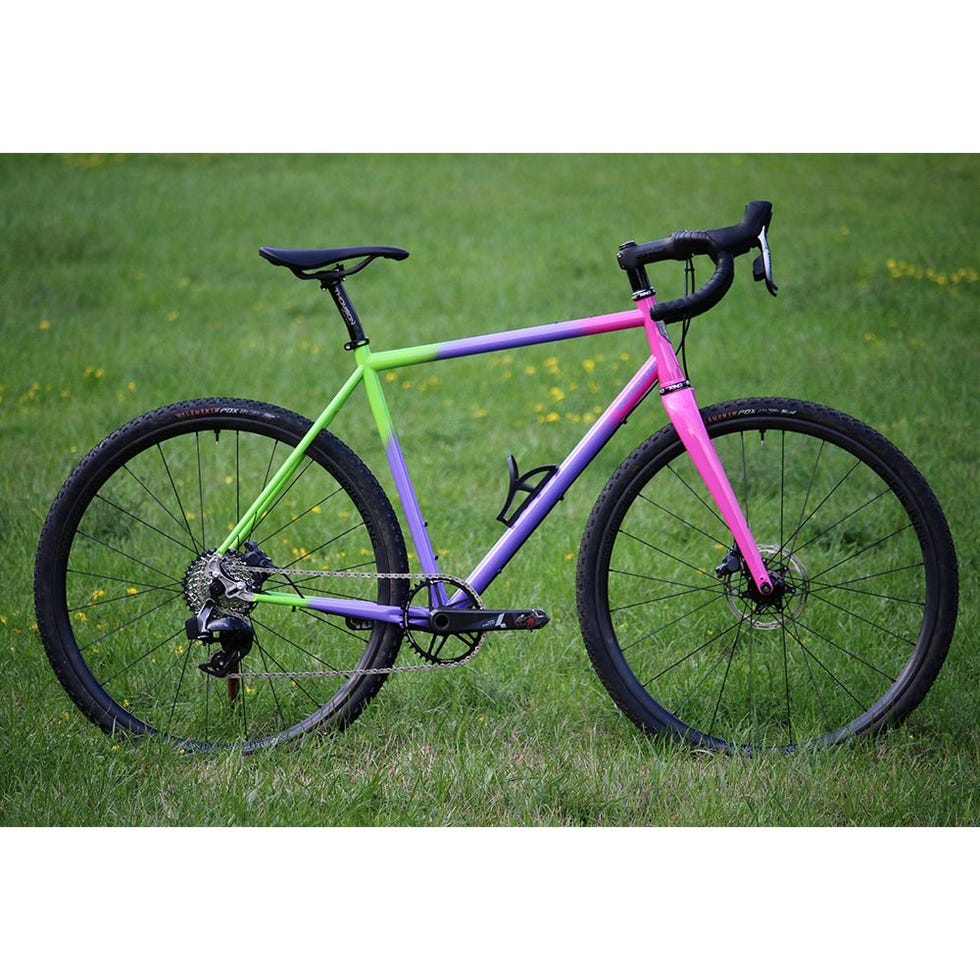In this detailed image of a bicycle, featuring a slim and minimal frame, the frame transitions through various vibrant colors: starting with green on the left side, it moves to purple and then to pink. This vivid blend gives the bike a dynamic, almost gradient-like appearance. The black components—the seat, handles, wheels, and gears—contrast sharply with the colorful frame. The bike is positioned in a large, grassy field peppered with small yellow flowers, creating a picturesque background. Interestingly, despite the lack of a stand, the bike appears to be standing freely. The focus is primarily on the bike, with the background slightly out of focus, giving it a professional or possibly AI-rendered effect. The bike resembles a 10-speed type or a mountain bike, adding to its sporty appeal, though there's some ambiguity about its origin due to its consistent tire branding.